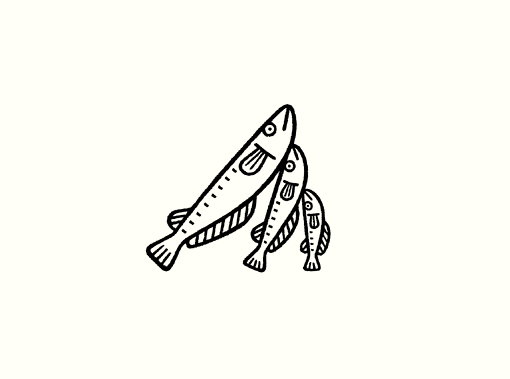This image features a simple yet detailed black line drawing of three fish set against a white background, all oriented with their heads pointing upwards to the right and their tails towards the bottom left. Each fish is depicted using minimalistic lines to represent their fins and tail, with intricately detailed folds and ribbing on the fins. The eyes are drawn as simple round circles positioned near the top edge of each fish, with a single dot in the center and a straightforward line for the mouth.

Starting from the bottom, the smallest fish is positioned perfectly vertical with its tail fin having two distinct lines. It also displays a small dorsal fin near its back and a larger ventral fin on its belly. Directly above and angled at around 30 degrees to the left, there is a middle-sized fish, approximately 30–40% larger than the smallest one. This fish aligns so its mouth touches the gill area of the fish beneath it, maintaining the same design elements as the smallest fish. At the top left, the largest fish is positioned at about a 45-degree angle, touching the middle fish in a similar manner. This largest fish is another 30% larger than the middle one, continuing the consistent design across all three, creating a visually cohesive arrangement with their noses touching and their bodies angled successively higher.